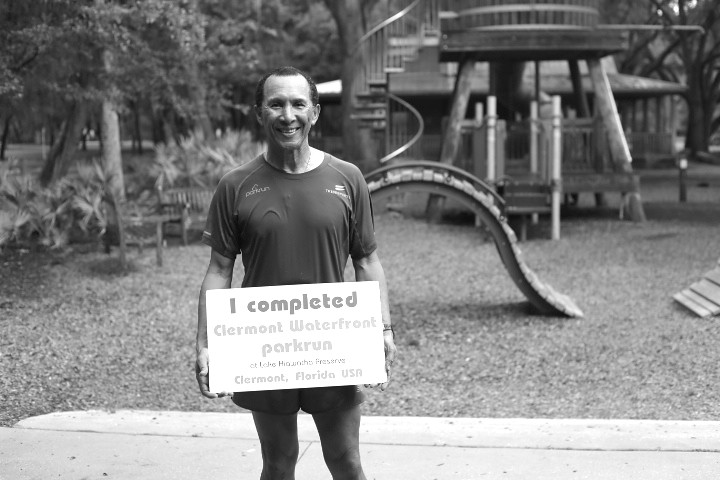In this black-and-white photograph, a man stands confidently at the Claremont Waterfront Park in Claremont, Florida, USA. Dressed in sportswear with a "Park Run" shirt, he proudly displays a rectangular white sign with gray text that reads, "I completed Claremont Waterfront Park Run." The man has a large smile on his face, revealing his teeth and exuding joy and accomplishment. He has very short, close-cropped hair and wears a watch on his left hand. The wooden boardwalk beneath his feet matches the light hues of the overall setting.

To the man's left, the backdrop features a cluster of trees with visible foliage. Behind him, partially obscured playground equipment indicates a lively, family-friendly area, including a slide, steps, and a platform that could resemble a treehouse for kids. Additionally, there appears to be a rounded building with steps further back. To the left of the man, a high-backed bench also sits amid the picturesque park landscape. The entire scene captures a moment of triumph and the serene beauty of the Claremont Waterfront Park.